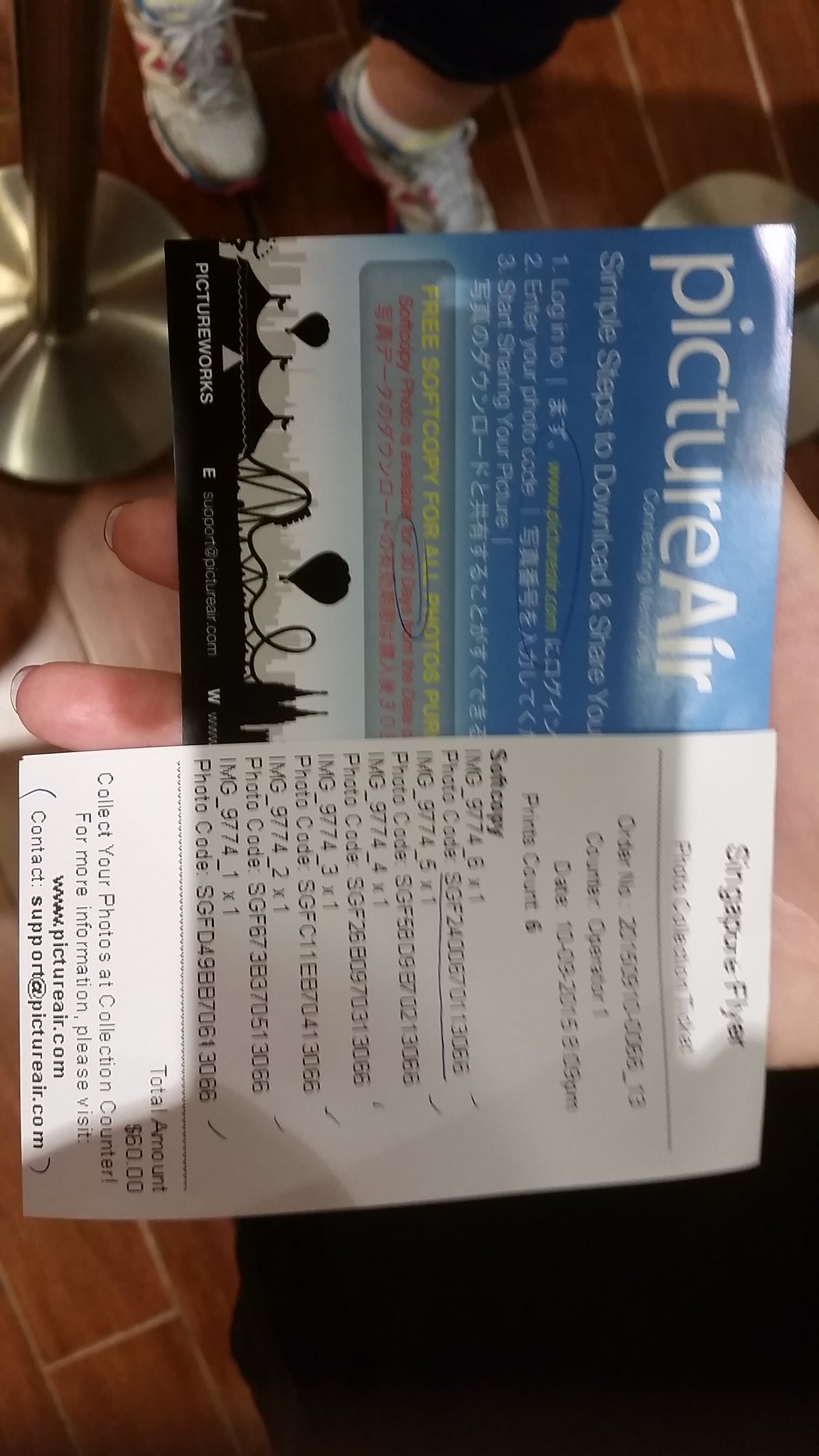The photograph, taken indoors from a top-down perspective, captures several intricate details. The ground, composed of brown tiles, sets a neutral backdrop. In the foreground, the photographer's hand is prominently displayed, holding two pieces of paper. The first paper is primarily blue with white text that reads "Picture Air," while the second is white with black text that says "Singapore Flyer." Next to the photographer stands another individual, wearing black pants and distinctive white and red tennis shoes. Between these two figures are metallic objects, likely fixtures or decorative items, comprising reflective silver bases with cylinders extending upward. The careful arrangement and sharp focus emphasize the contrast between the papers, the attire, and the metallic objects, creating a visually compelling and contextually rich image.